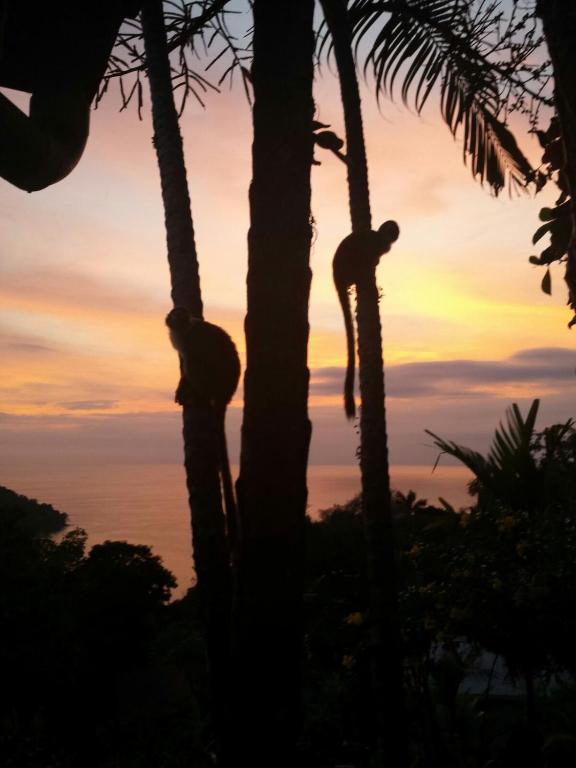This captivating image captures the essence of a tropical rainforest at sunset. Bathed in hues of pink, yellow, and purple, the sky transitions to pale shades of gold, orange, and gray as the last rays of sunlight fade. The scene is set from a vantage point that appears to overlook an ocean, creating a strikingly serene backdrop. Dark silhouettes of trees, especially thin, towering palm trees, dominate the foreground. Within these trees, two monkeys are visible, their tails hanging down as they climb or rest, seemingly curious about the photographer. The contrast between the vibrant sunset sky and the darkened jungle enhances the mystical allure of this tropical paradise.